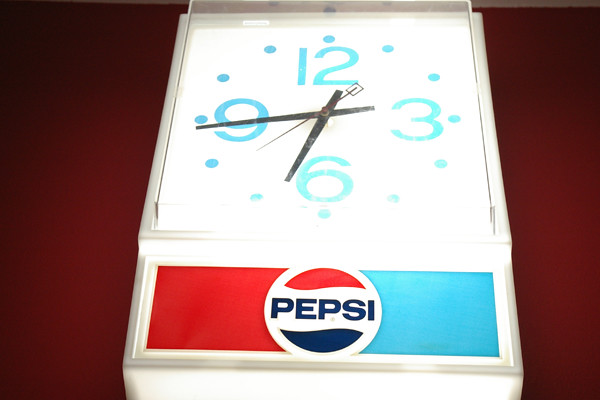An illuminated Pepsi-themed wall clock is mounted against a maroon, orangish-maroon colored wall, possibly in a house or a restaurant. The clock features a white background on its face with a prominent Pepsi logo positioned below the center. This logo boasts the classic design, with the top half in red and the bottom half in blue, sandwiching the word "Pepsi" in blue text on a white backdrop. The left side of the logo is bordered by a red section, while the right side is bordered by a blue section. The clock's numerals for 12, 3, 6, and 9 are displayed in light blue, while smaller light blue dots mark the remaining hours. The hour, minute, and second hands are colored in a blackish-grayish hue, completing the clock's functional elements.